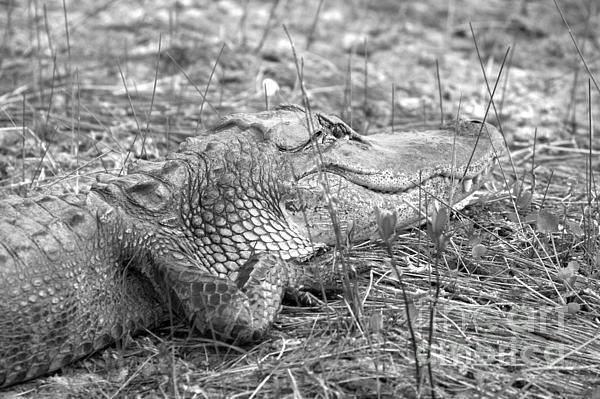In this black-and-white, grayscale photograph, an alligator lays on the ground, camouflaged among dried grass and scattered twigs. The image captures the creature from an angle slightly behind and to the side, showcasing its textured scales and one dark eye. Its mouth is partially visible, revealing some sharp teeth. The alligator's right front arm is positioned near its neck, and the head is turned to the right, indicating a resting pose. The background consists solely of the dry, twig-filled terrain with no water or sky visible. A watermark appears in the right-hand corner, though the text within it is indiscernible, further emphasizing the minimal context provided by the scene.